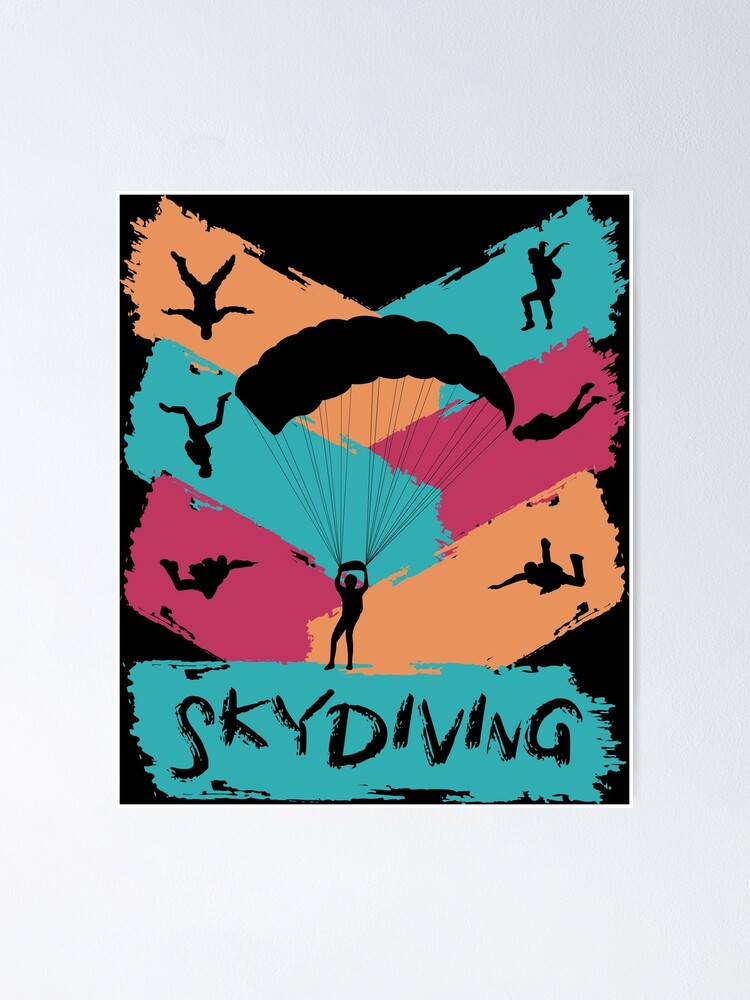This striking poster, framed with a grayish white matte, is designed to promote skydiving. It is taller than it is wide and features a vibrant and dynamic artwork with a black background. The word "SKYDIVING" is boldly displayed in large capital black letters against a teal backdrop at the bottom of the poster. The poster depicts a black silhouette of a skydiver navigating a small steerable chute, surrounded by broad, painted-looking bands in vivid shades of hot pink, cyan, and a peachy-orange. These bands add a colorful, almost abstract element to the image and intersect with each other. Within these color bands are various black silhouettes of skydivers in different positions – some soaring, some with bent legs, and some in freefall – capturing the exhilarating experience of skydiving. The overall effect is a visually engaging and colorful piece, clearly meant to be hung on a wall to entice viewers with the thrill and adventure of skydiving.